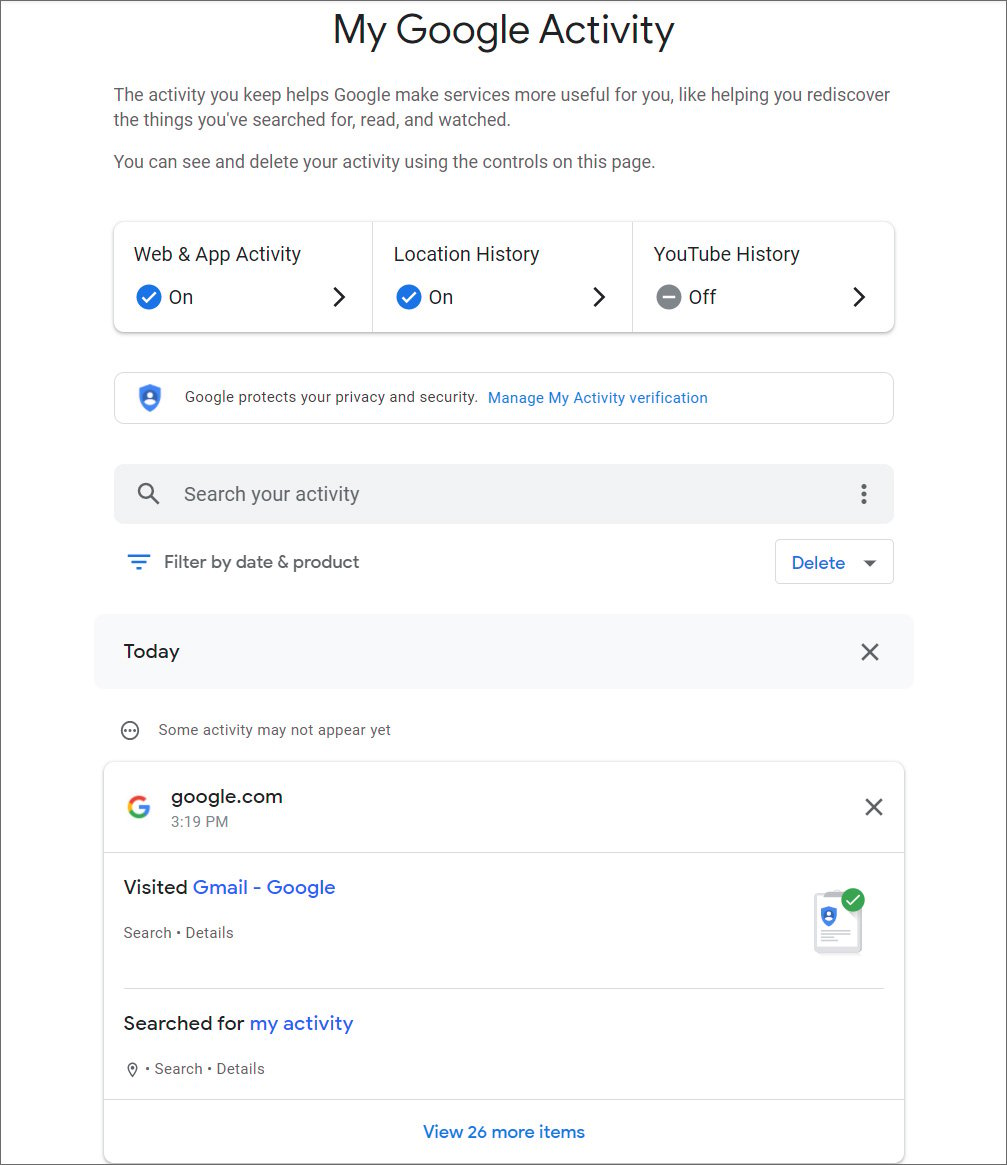On the "My Google Activity" page, users can manage the data that Google collects to enhance its services. This page provides a transparent overview, allowing individuals to rediscover things they've searched for, read, and watched. Users have the ability to see and delete their activities using various control options available on this page. Key features include toggles for Web and App Activity, Location History, and YouTube History. In this instance, Web and App Activity, and Location History are enabled, whereas YouTube History is disabled. Further down the page, there's a search bar to explore specific activities and filters to narrow results by date and product. The recent activity section highlights today's actions, including visiting Gmail and searching for "My Activity." It notes that some recent activities might not appear immediately. At the bottom of the page, a button reveals an additional 26 items, showcasing a comprehensive log of browser activities while signed into the Google account.